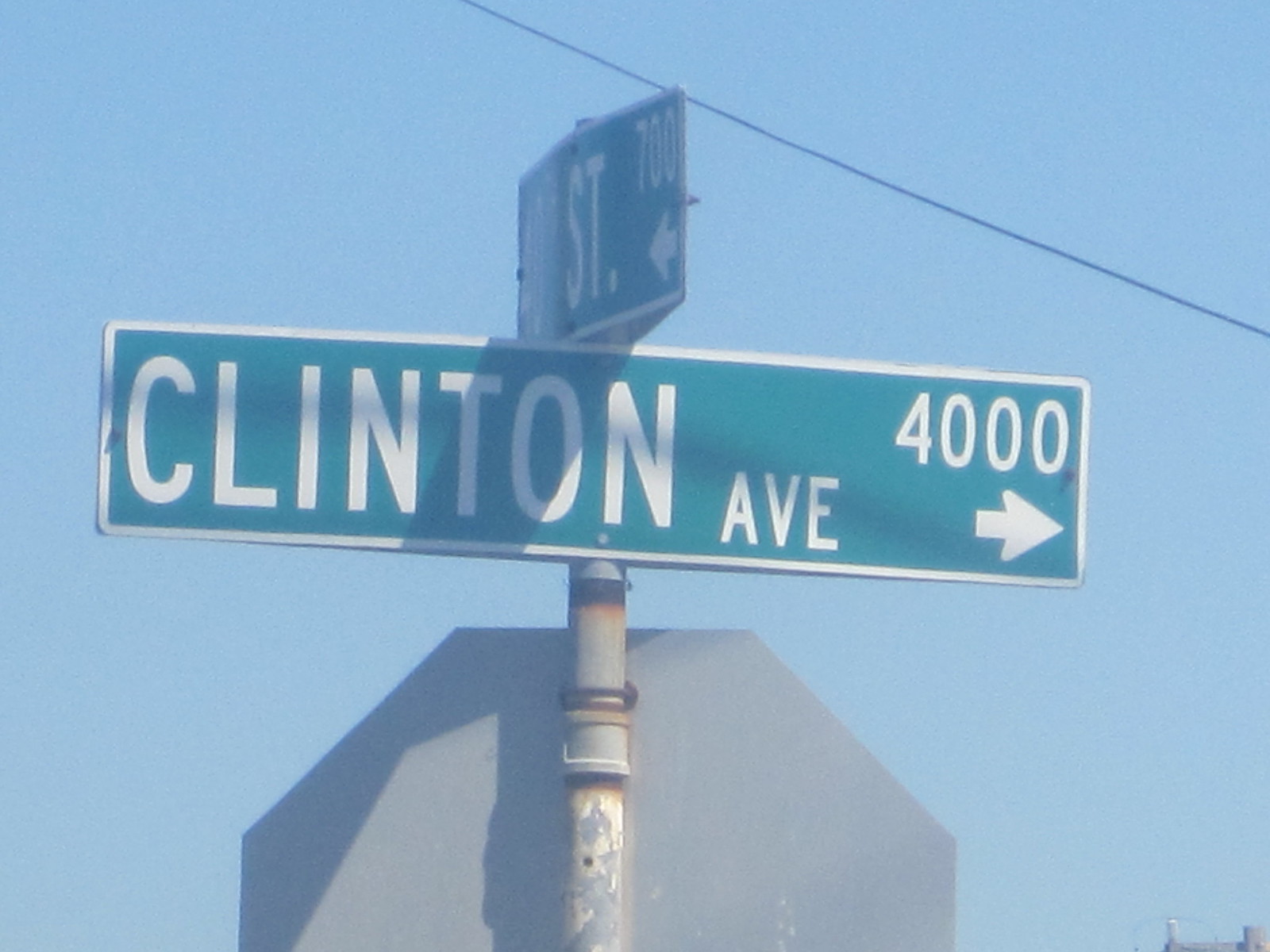This image captures a tightly framed intersection sign mounted on a rusted, crusty silver pole. The primary focus is on a green street sign with white lettering that reads "Clinton Ave" and "4000," accompanied by a right-pointing white arrow. Mounted above it is another sign, partially visible, indicating "ST" and "700," with an arrow pointing to the left. The top portion of a stop sign, viewed from the back, reveals a gray metal hexagon shape behind the pole. A single power or telephone line runs diagonally from the top center towards the upper right corner, set against the backdrop of a bright, cloudless blue sky. A hint of a couple of buildings can be seen in the lower right-hand corner, adding context to the urban setting. The details emphasize the age and weathering of the metal brackets and pole, highlighting the dark brown rust spots.